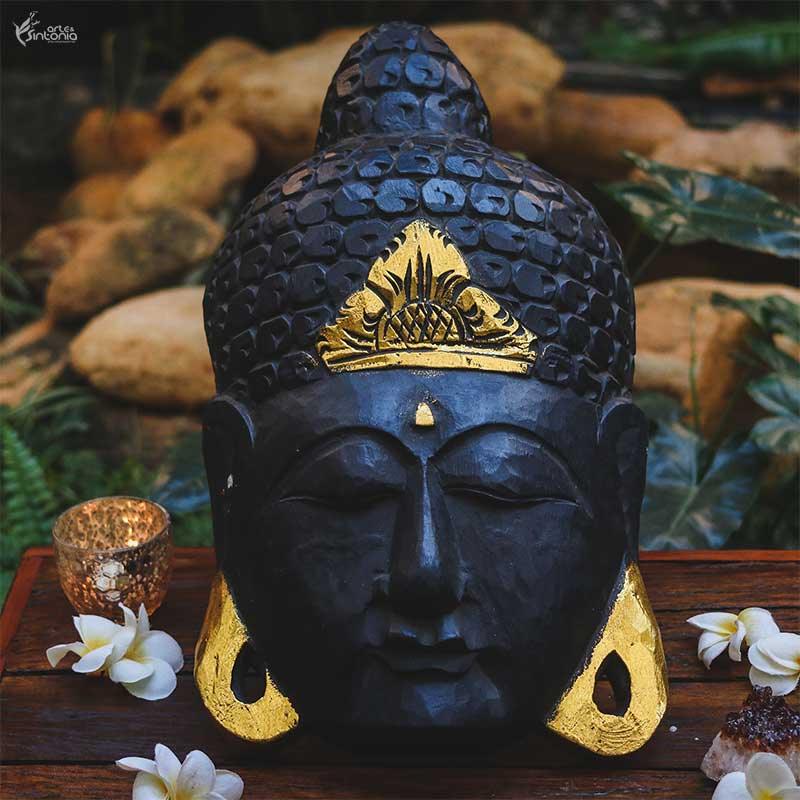This detailed photograph showcases a black Buddha head sculpture, possibly crafted from wood or metal, exuding a serene and meditative aura with closed eyes. The sculpture is intricately decorated, featuring gold-painted elements, including elongated earlobes or earrings, a distinct third eye area, and a triangular gold design on its forehead. It wears a distinctive headdress adorned with raised circular patterns and a central gold embellishment resembling a pineapple. The Buddha head statue is positioned on a red wooden table, accompanied by white plumeria flowers with yellow centers and a translucent golden candle holder. The backdrop is a blurred, tranquil arrangement of green leaves, ferns, and brown rocks, which enhances the serene focus on the beautifully adorned Buddha head sculpture.